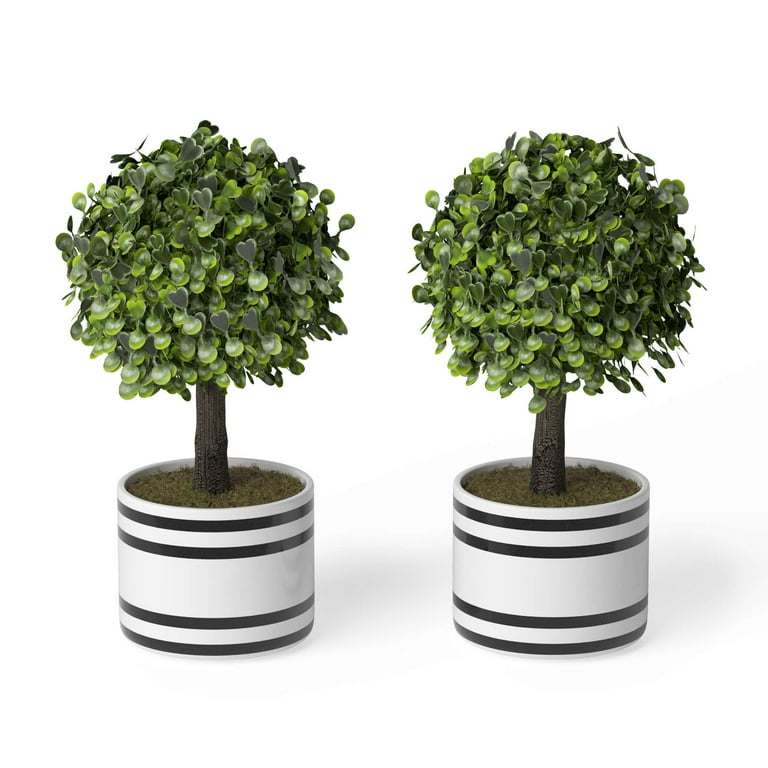The image shows two identical miniature tree-like plants, each contained in an identical circular white pot with distinct black stripes—two close-together stripes near the top and bottom, separated by a wide white area. The dark brown trunk of each plant rises from dark brown soil, leading to a dense, well-groomed canopy of leaves shaped into a solid, rounded top. The foliage is a mix of heart-shaped and round leaves, with the heart-shaped ones being very dark green and the round ones lighter green. These two pots are placed side by side in a horizontal layout with no visible background, making the plants and pots the central focus.